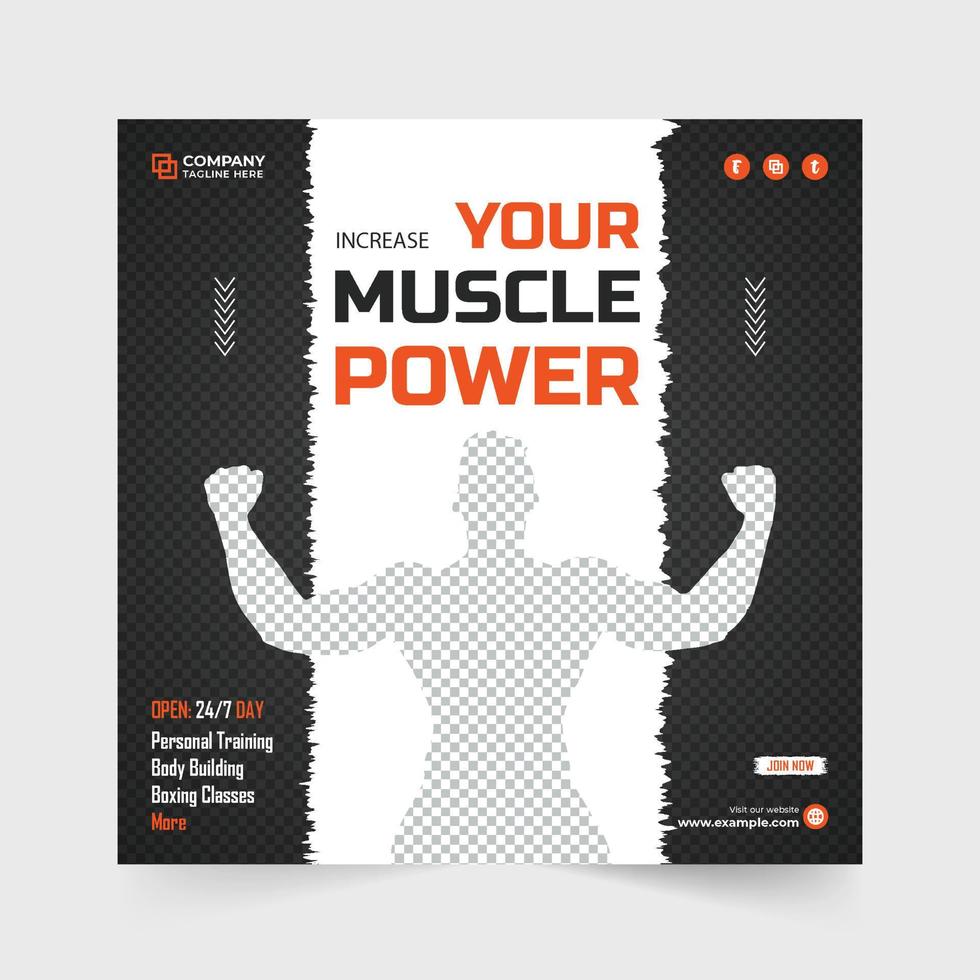The image appears to be a promotional ad for a gym, likely designed as a CD cover. It features a central white rectangle with rough, torn paper-like edges, flanked by black sides. At the top left of the white area, it says, "Increase Your Muscle Power," with "increase" and "muscle" in black and "your" and "power" in large orange font. Below this text is the gray and white checkerboard silhouette of a muscular person flexing with both fists raised. On either side of the white rectangle, the text reads, "Open 24-7 daily personal training, bodybuilding, and boxing classes." The top left corner of the black background includes placeholder text "company tagline here" in white, accompanied by two interlocking red squares. The top right corner features social media icons: an "F," the interlocking red squares again, and a "T." Additionally, the bottom left corner reads, "visit our website www.example.com," with an orange circular globe icon beside it. The bottom right corner features a torn paper-like area with orange text that says, "Join Now." The entire design suggests a template for gym advertising, allowing customization for specific taglines and website details.